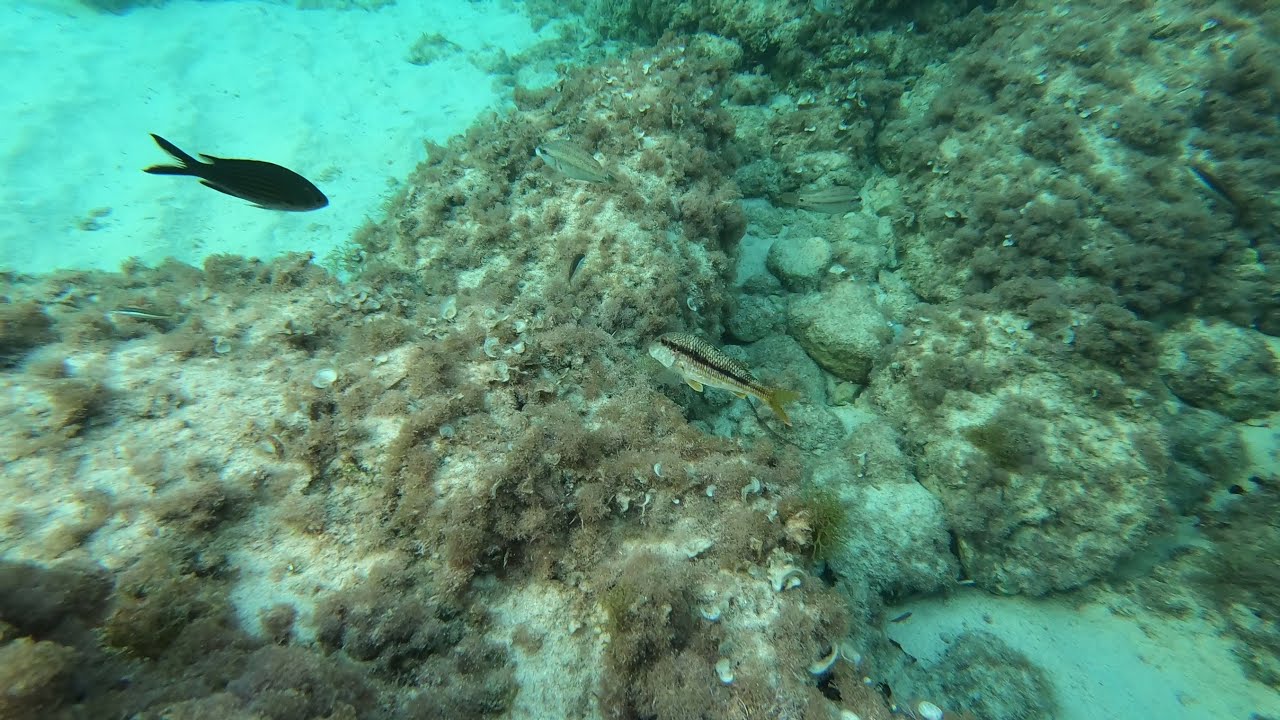In this color photograph, a landscape-oriented underwater scene showcases a clear, light bluish-green aquatic environment reminiscent of an aquarium. The sandy ocean floor, tinted blue by the water, is visible in the upper left corner, seamlessly transitioning to brown and white coral interspersed with a rocky ocean bed that extends from the lower left corner to the top right. Scattered throughout the scene are numerous algae-type plants and shells. Prominently featured in the image are at least four slender fish. In the center of the sandy area is a medium-sized black fish, possibly shadowed, facing three other fish near the coral. These other fish exhibit varying colors: one with a horizontal black stripe, another with a tannish color and golden fins, and a silverish fish with brown specks. The photograph's clear and detailed realism captures the serene and vibrant life of the underwater world.